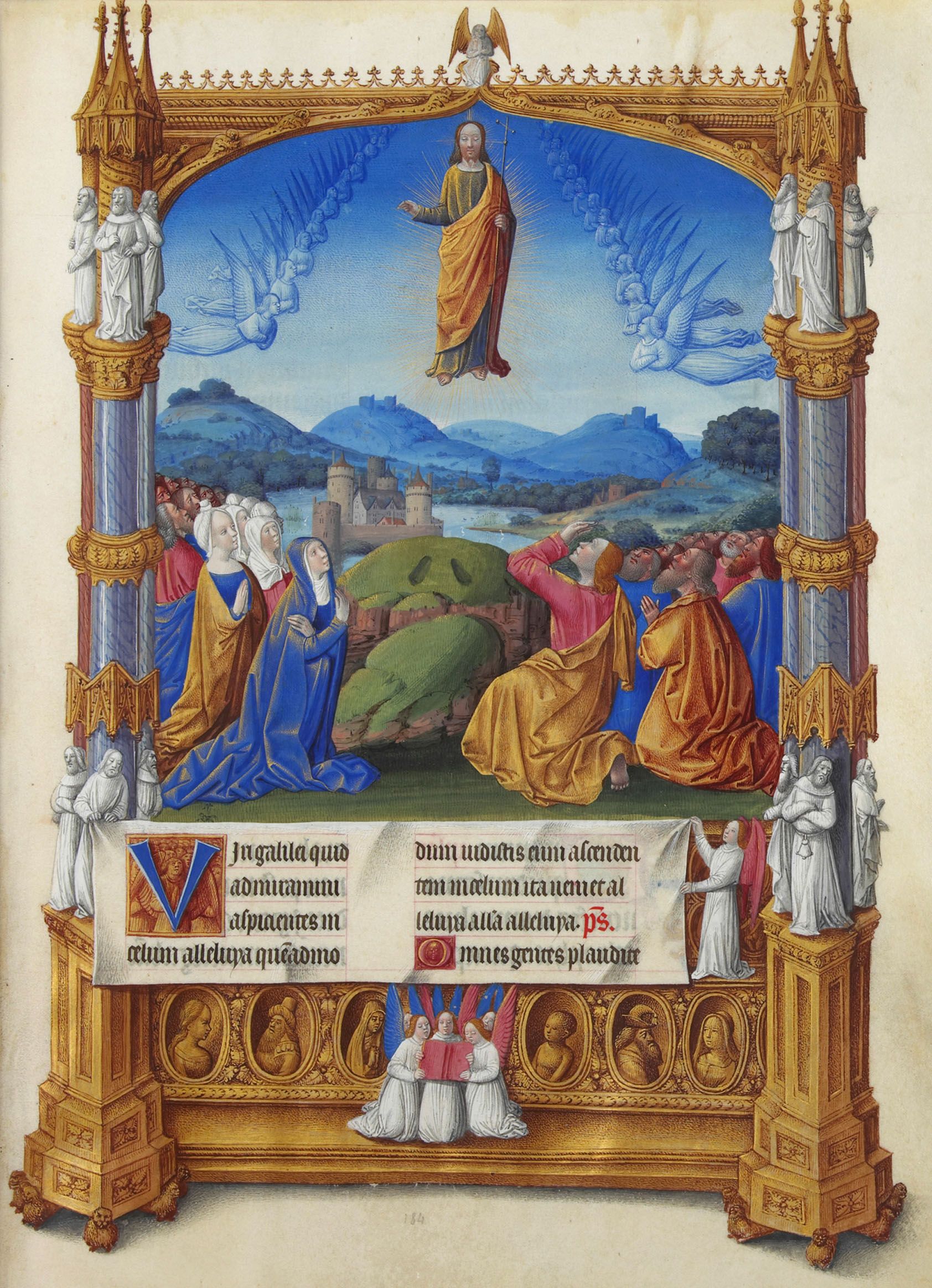The image depicts an elaborate and detailed religious painting often found in a church. Central to the scene is Jesus, depicted rising above a group of followers kneeling on the ground, looking up at him in devotion. He is adorned in a brown robe that drapes over his shoulders with his right hand extended outward. The background features a sky of a blue hue with mountains and a castle, adding depth and context. 

The ornate frame surrounding the painting is intricate and gold-toned, accented with tower-like spikes on the sides and small figurines, possibly saints, inset into the bottom. A bridge-like element connects these towers at the top, while the base of the frame includes several oval-shaped miniature depictions, such as three praying monks. Above these figures, there is a white scroll with Latin script, notably featuring a large letter "V" on the left.

Overall, the painting's medieval, two-dimensional style and its detailed framing create a profound religious atmosphere, capturing a moment of divine ascension and reverence among the followers.